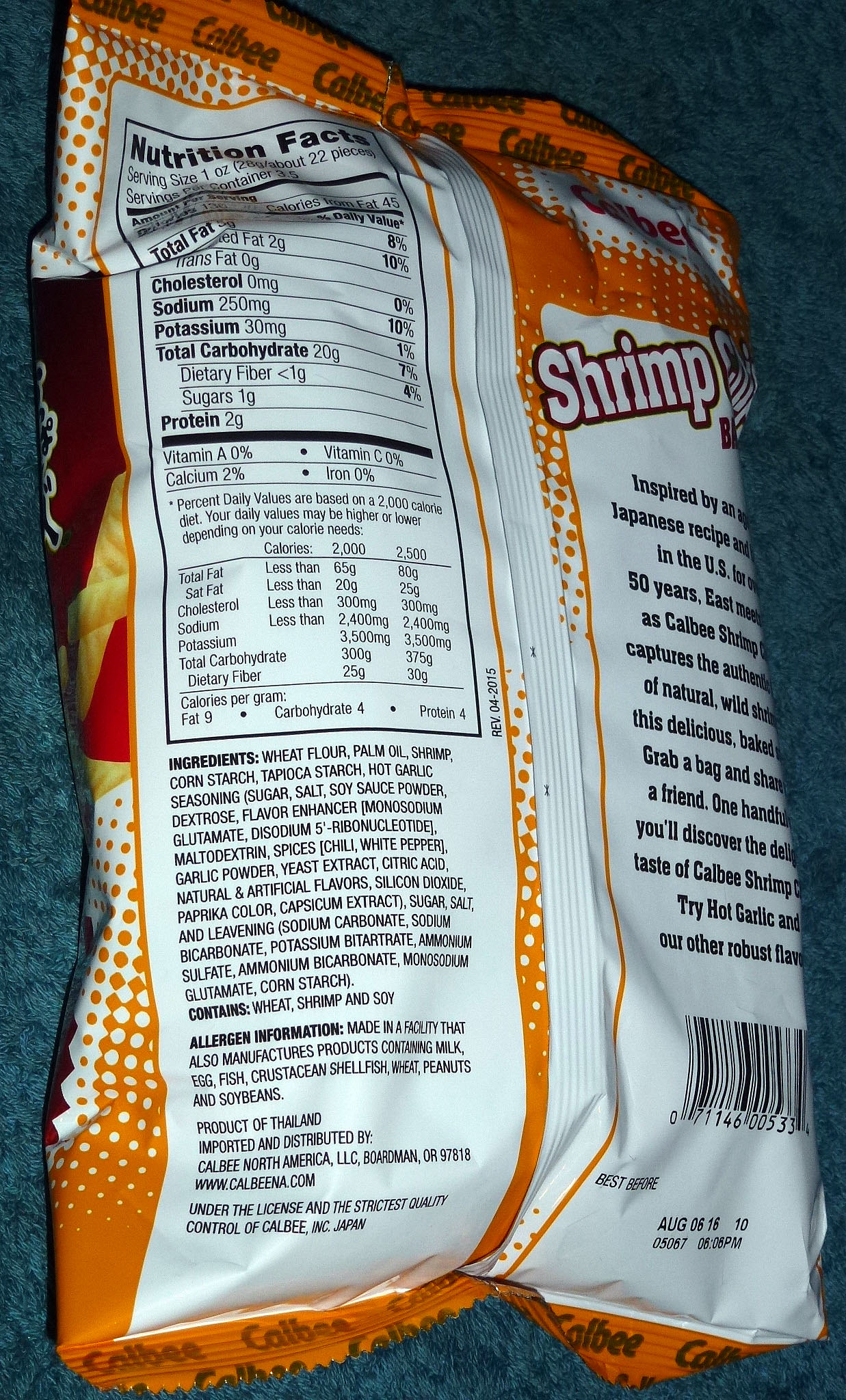The image depicts the back of an orange and red package of shrimp crackers, resembling Asian shrimp snacks that look like crispy french fries. Prominently on the left side, a white rectangle details nutritional information, including metrics like total fat, cholesterol, sodium, potassium, total carbohydrates, dietary fiber, sugars, protein, vitamin A, calcium, vitamin C, and iron, alongside daily value percentages. Beneath the nutrition facts, separate sections list ingredients and allergen information. The word "shrimp" appears in bold white letters outlined in black on the upper right side, accompanied by a brief background story about the product. The bottom of the package features a black barcode and an expiration date. The overall design includes an orange border at the top and bottom, and the brand name "Kyle B." is visible in black text. Hints of the colorful front design and images of the shrimp crackers can be seen from the side.